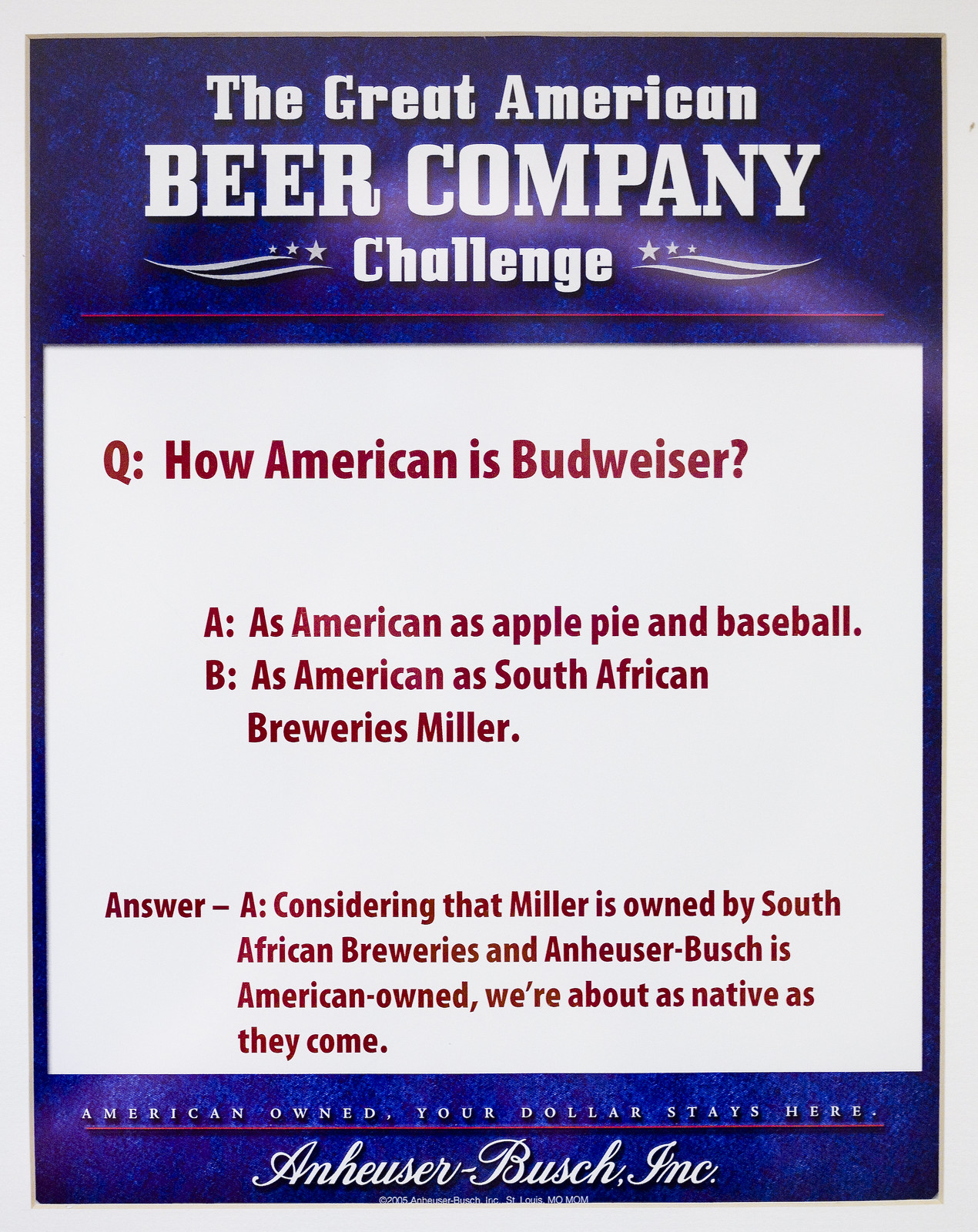This detailed flyer is for "The Great American Beer Company Challenge," set against a deep blue background with a combination of dark blue and bright blue highlights, peppered with black specks. The top portion of the flyer prominently features three large white lines of text that read: "The Great American," "Beer Company," and "Challenge." 

At the center of the flyer, a white rectangle houses multiple lines of bold red text, formatted as follows: 

- "Q: How American is Budweiser?"
- "A: As American as apple pie and baseball."
- "B: As American as South African brewery’s Miller."
- "Answer: A. Considering that Miller is owned by South African breweries and Anheuser-Busch is American owned, we're about as native as they come."

The bottom of the flyer underscores its main message with the slogan "American owned, your dollar stays here," indicating a sponsorship by Anheuser-Busch Inc. The entire layout is framed by a light gray border, emphasizing the flyer’s professional and compelling design.